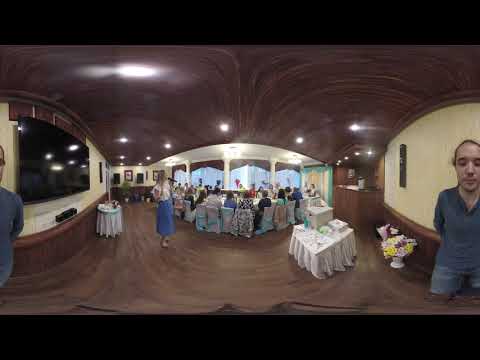The image portrays a lively social gathering that appears to be set in a brown-ceiling and brown-floor venue, possibly a banquet hall or restaurant. Central to the scene is a long table adorned with white tablecloths, around which numerous adults are seated, suggesting a formal event like a wedding reception, birthday party, or brunch meeting. The chairs, draped in fabric that resemble quilt patterns, add to the festive atmosphere.

To the left, a woman in a white blouse and blue skirt stands holding a microphone, indicating she might be singing or speaking to the guests. To the right, a younger man, possibly in his 20s, is seen wearing a blue shirt and blue shorts, with his hair neatly tied back in a ponytail. Another man, in gray shirt and shorts, stands toward the right of the frame.

In the background, attendees are seated around circular tables, one of which appears to have a significant item or symbol, like a cross. The presence of ceiling lights and the overall ambiance hint at a well-orchestrated event. The atmosphere is vibrant yet intimate, befitting a noteworthy celebration.